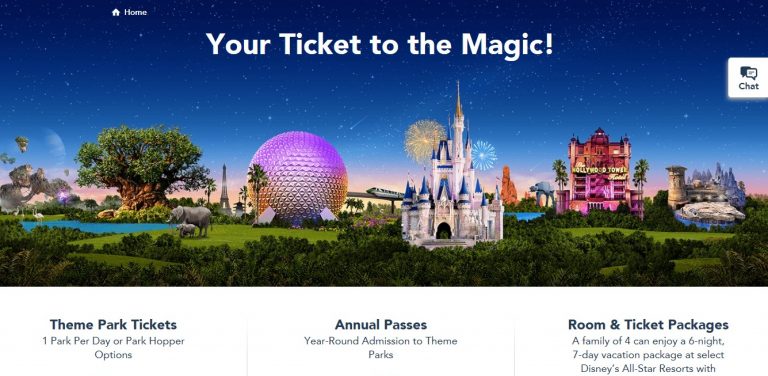In this vibrant and enchanting Disney promotional image, a variety of delightful elements converge to capture the magic of a Disney vacation. The bottom section of the image features a white background on the left, transitioning into dark blue hues. Text in this section highlights various offers: "Theme Park Tickets," providing options for one park per day or park hopping; "Annual Passes," offering year-round admission to the theme parks; and "Room and Ticket Packages," detailing a vacation package for a family of four to enjoy a six-night, seven-day stay at select Disney's All-Star Resorts.

Against the backdrop of a nighttime sky adorned with white stars, a prominent white text exclaims "HOME" in the upper left corner. In the center, bold text reads, "You Are Ticket To The Magic!" with the words "You," "Ticket," "The," and "Magic" capitalized and emphasized. 

A white box with black text labeled "Chat" is positioned nearby. Central to the image is a depiction of the iconic Disney castle, predominantly white with blue-tipped towers, set against a backdrop of colorful fireworks - gold and yellow on the left side and blue on the right.

The image also features notable Disney landmarks: the spherical Epcot Center, partially white at the bottom and black at the top, the Eiffel Tower, and natural elements such as elephants and flamingos by a water body with a tree. Additionally, the Disney tram, known for transporting visitors through the parks, is depicted, completing the scene with a touch of practicality amidst the fantasy.